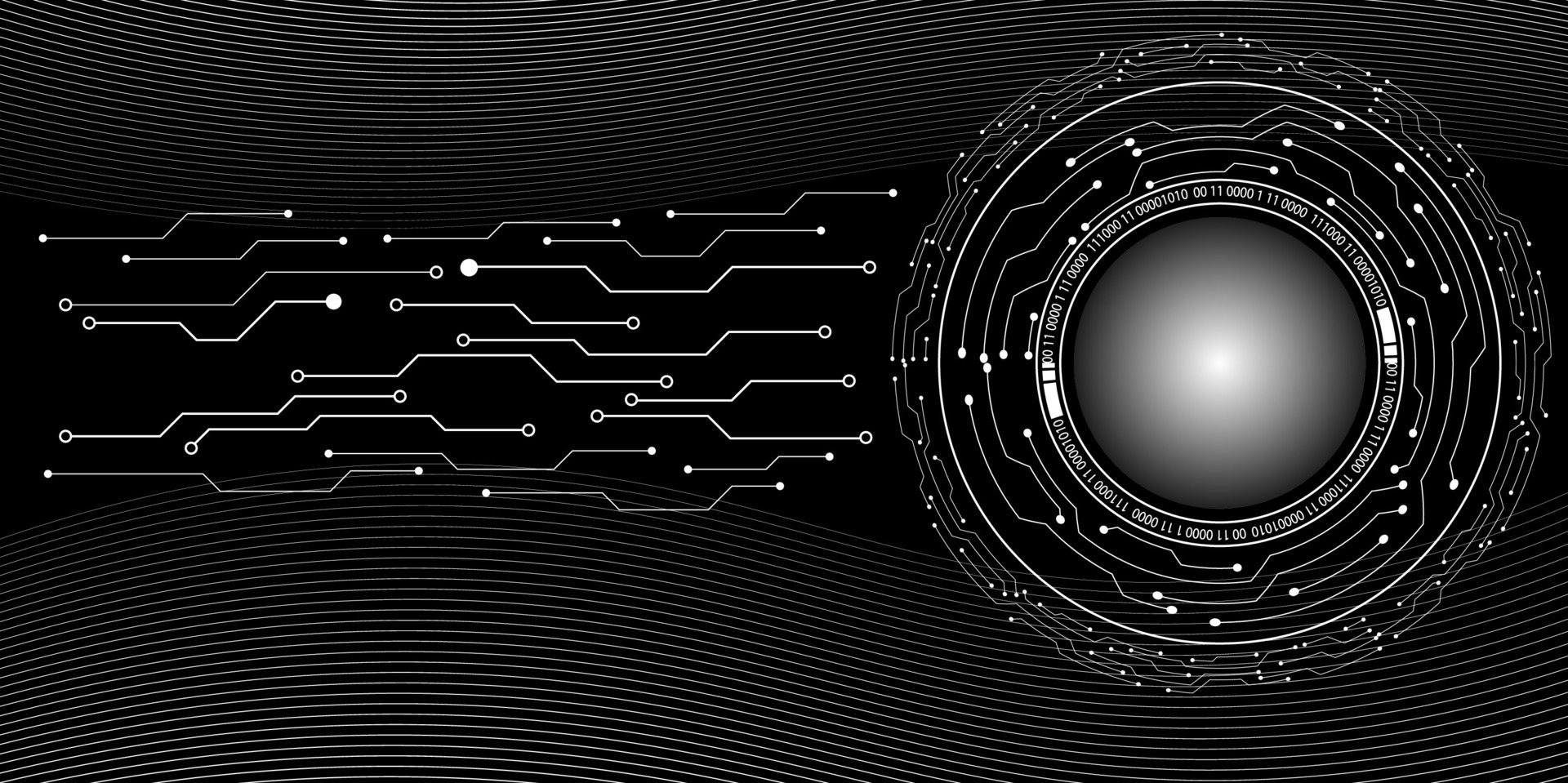The image is a highly detailed, black and white computer-generated design with a complex, symmetrical structure. At its center-right, there is a luminous white sphere surrounded by a series of concentric circles. The innermost circle is adorned with binary code—ones and zeros—forming a ring around the bright core. Extending from these circles are various geometric and abstract line shapes, each highlighted with small white dots at the ends, reminiscent of a computer chip's intricate circuitry. The left side of the image features more of these chip-like lines, primarily oriented horizontally. The entire image is framed by dark wavy lines that gradually brighten towards the edges, creating a reflective pattern. The overall impression is that of a technical illustration or computer animation, with elements that suggest the inner workings of electronic components or a futuristic design.